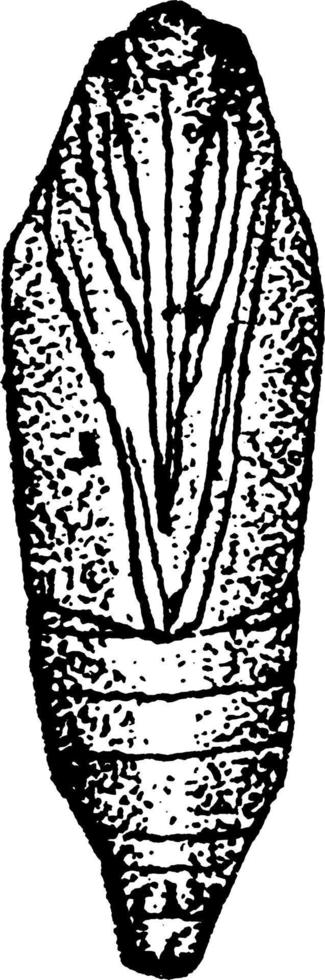This is a detailed black and white line drawing of an oblong object, reminiscent of a cocoon or a small fat cigar. The drawing is done in black ink on a white background and features heavy black lines with pointillist-style shading, giving it a textured appearance. The object, which resembles a carved stone or an archaeological artifact, has horizontal striations towards the bottom and longitudinal striations that extend from the center towards the top. The shape is extended and oval-like, with vertical lines running down its center for about two-thirds of its length. Five horizontal lines are evenly spaced across the bottom section. The surface detailing of the object, filled with black dots and squiggles, suggests a rough texture, similar to an insect larva or potentially a stone hammer.